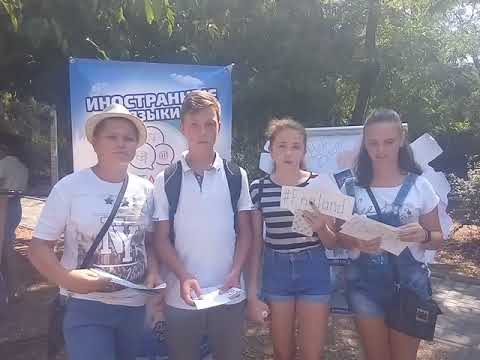In this bright outdoor image, four young people stand in a line, looking forward. From left to right, the first person is wearing a white graphic t-shirt with 'NY' in white letters, blue jeans, and a white fedora. A black sack hangs across their shoulder. Next to them is a boy in a white polo shirt, carrying a black backpack and wearing gray pants. Following him, a girl dons a white and black striped shirt with short blue jeans, holding a sign that reads "#England" in her hand. The last person is a girl wearing short blue coveralls over a white t-shirt, with a black purse slung over her shoulder. Behind them is a sign featuring the backwards letters "N-H-O-C-T-P-A-H" and other designs underneath. The background is filled with lush foliage, including trees and leaves, and to the extreme left, the back of another person is partially visible, facing away from the main group.